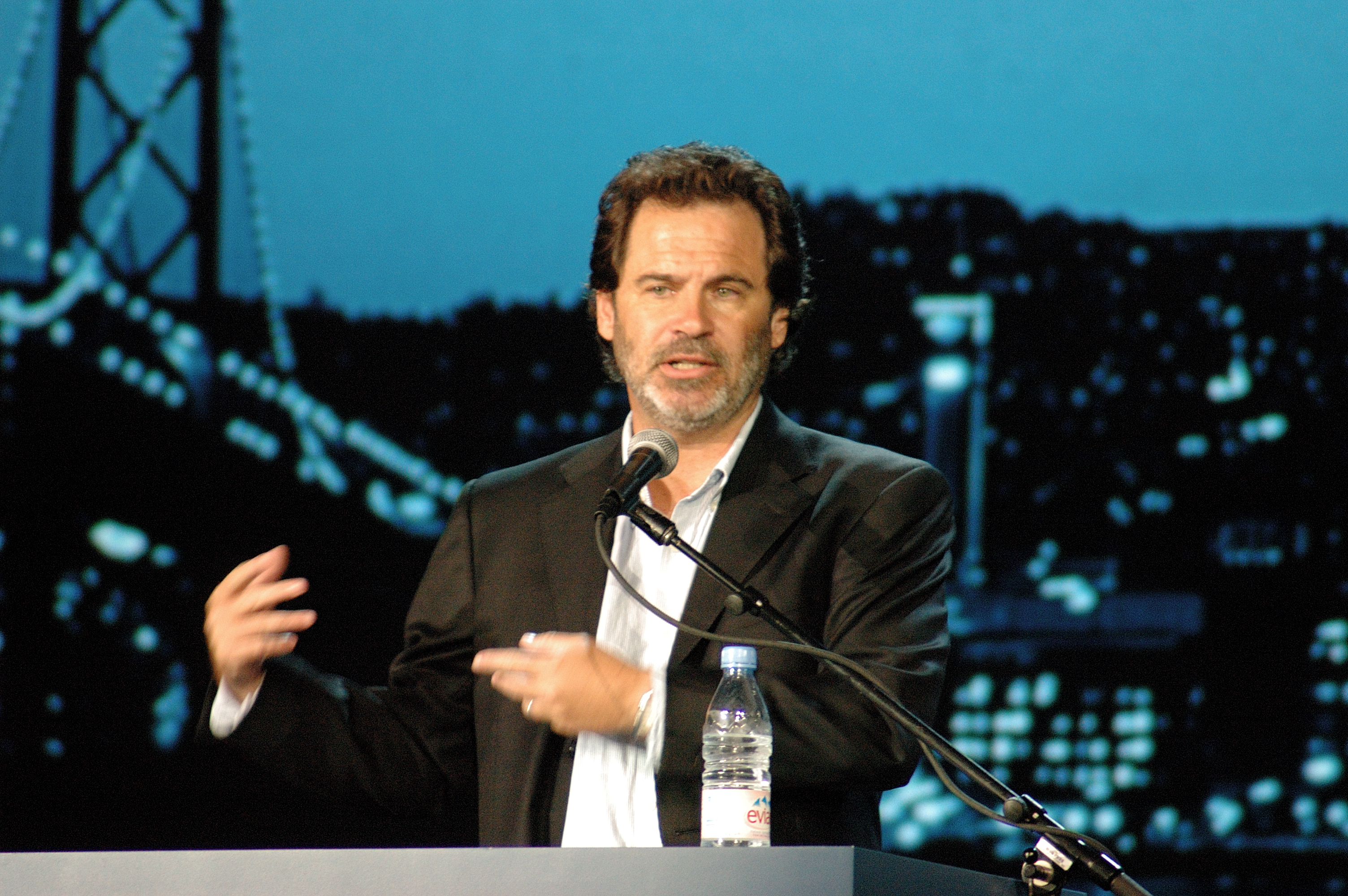In this horizontally oriented photograph, comedian Dennis Miller is captured giving a talk, likely as part of a political or stand-up engagement. He stands at a gray, or possibly silver, lectern equipped with a prominent microphone extending toward his mouth. His mouth is slightly open, suggesting he is in the midst of speaking, and his hands are animated in front of him, adding expressiveness to his speech. Dennis, known for his sharp wit and political humor, is dressed in a black suit coat over a white button-down shirt, notably without a tie. 

On the right side of the lectern, a partially consumed plastic Evian water bottle is visible. Dennis sports dark brown hair and a scruffy mix of brown and gray facial hair, giving him a rugged, casual appearance. The background features an abstract depiction of a city skyline with elements suggestive of the Golden Gate Bridge angled diagonally above his left hand, and dark blue buildings with light blue windows to his right. The overall scene suggests a late-night talk show or a formal speaking engagement, blending the look of a televised set with an urban nightscape backdrop.